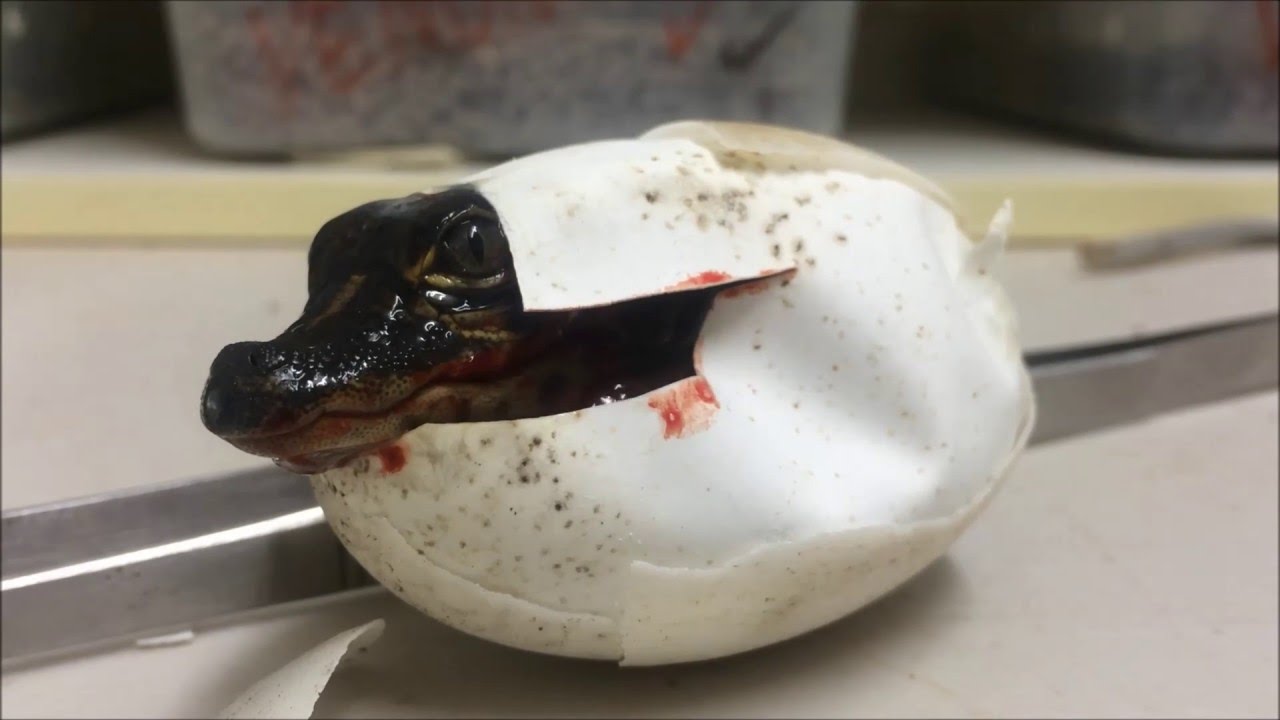This photograph vividly captures a baby crocodile hatching from a soft, white egg with black speckles. The tiny reptile's head, adorned with large, cautious eyes sporting the distinctive vertical irises, pokes out from a rupture in the egg. Red fluid decorates the edges of the soft eggshell, perhaps signaling the recent break through. The scene is set on a white countertop or table in what appears to be a laboratory environment, accentuated by a silver railing next to the egg. In the background, a yellow shelving unit and plastic containers are visible, adding context to the experimental setting. The little crocodile, central to the image, looks endearingly surprised as it takes in its new surroundings.